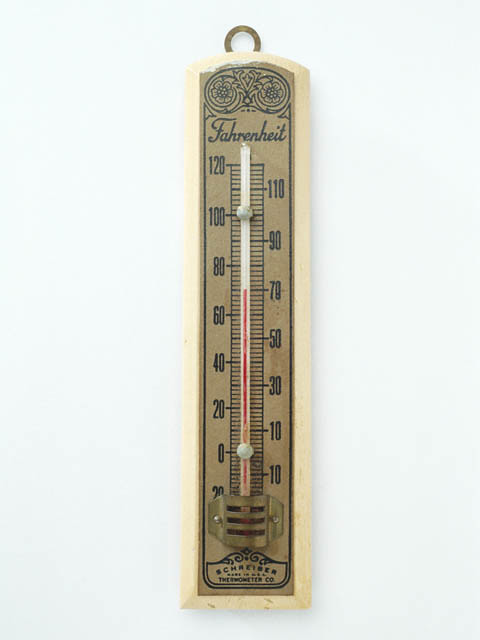This image features a white wall adorned with a classic thermometer. The thermometer itself is designed with a white casing and is equipped with a small circular hook at the top for wall mounting. It features a brown background and elegant floral designs at the upper section. The word "FAHRENHEIT" is prominently displayed, written in a formal typeface with a white underline. Within this underline, a red line indicating the temperature reaches up to 70°F. 

On the left side of the thermometer, temperature markers are listed in descending order: 120, 100, 80, 60, 40, 20, and 0 degrees Fahrenheit. A metallic piece is also visible, serving as part of the thermometer's measurement mechanism. On the right-hand side, the temperature markers read 110, 90, 70, 50, 30, and 10 degrees Fahrenheit. Below the thermometer, there is an inscription that reads "SCHCENEBER," adding a further element of detail to this utilitarian yet decorative piece.